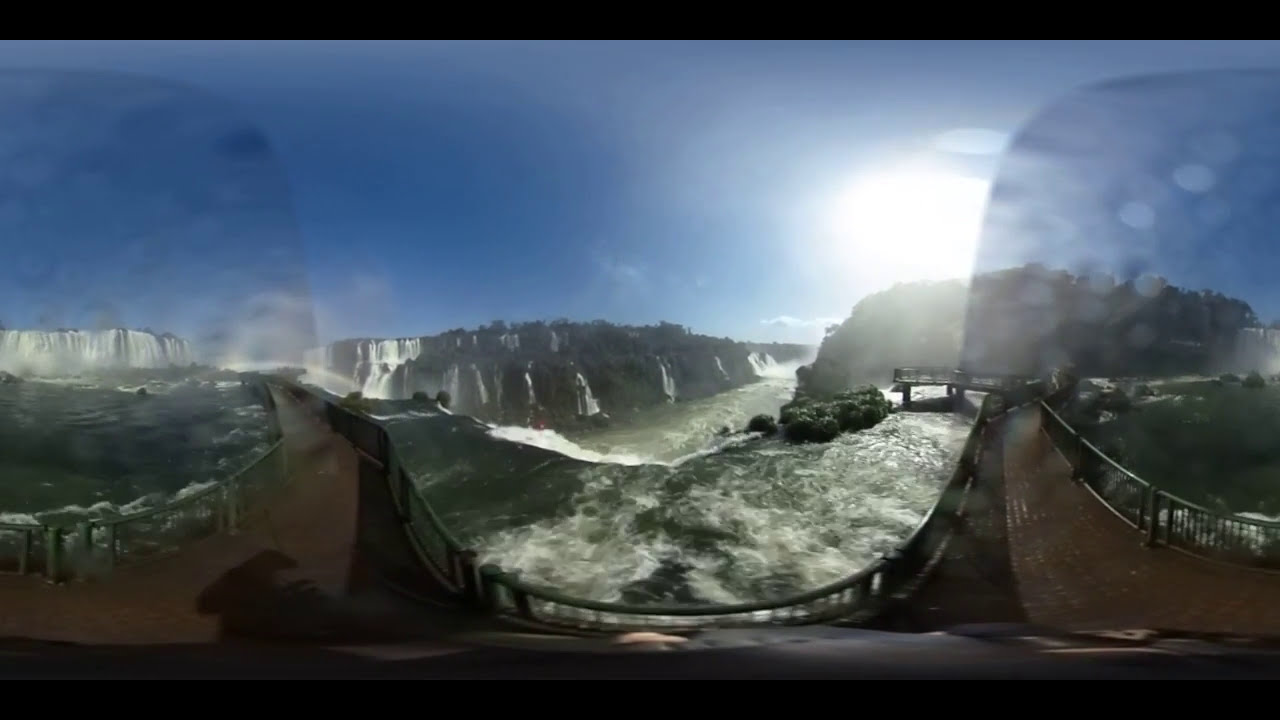This image is a panoramic shot, possibly using a fisheye lens or VR technology, of an area saturated with cascading waterfalls. The water flows down multiple cliffs on either side of the viewer's perspective, creating a scene of gushing rapids and frothy white caps. In the center of the picture, there's a brown brick footpath forming a U-shape, running elevated over the water with guardrails for safety. This pathway appears to be occasionally cut off due to the panoramic or 360-degree imaging, but it offers a closer view of the waterfalls. Along the path and in the surrounding area, you can see trees growing on rocky outcroppings amidst the falling water, adding to the natural beauty of the scene. The water varies in color, appearing blue closer to the center of the image where the falls are most active, and turning greener towards the bottom. Additionally, some black framing, in the form of small rectangles, is present at the top and bottom of the image, likely artifacts from the digital imaging process. The entire scene is devoid of human presence, emphasizing the untouched, wild nature of the cascading waterfalls and the lush, green landscape.